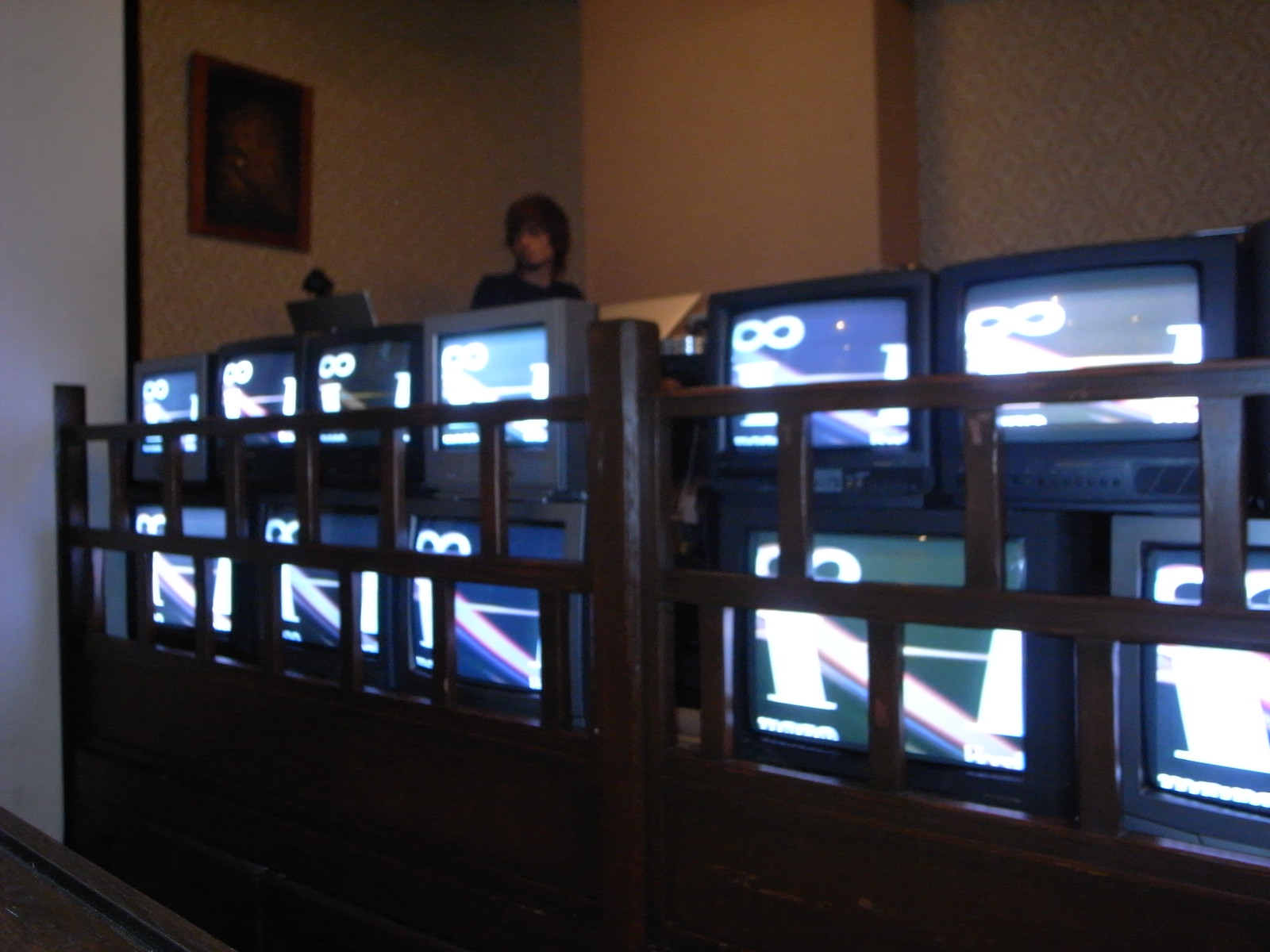The image shows a room with a rectangular layout, featuring a wall of televisions set behind a wooden, grated divider. The divider, resembling a fence made of brown vertical and horizontal rods, partially obscures the view of the TVs. The television wall comprises roughly twelve older, cathode ray tube (CRT) monitors of varying sizes and colors, arranged in two rows – six smaller monitors on top and six larger ones below. All the screens seem to be displaying the same program. 

Behind this setup stands a man with medium-length brown hair swooped to the left. He is focused on a silver laptop. The background reveals walls adorned with white and gray decorative wallpaper, and there is a painting with a brown frame hanging to the left of the man. The entire scene is somewhat dimly lit, adding to the intrigue of the setting, which could be an internet café, a store display, or an office divider.